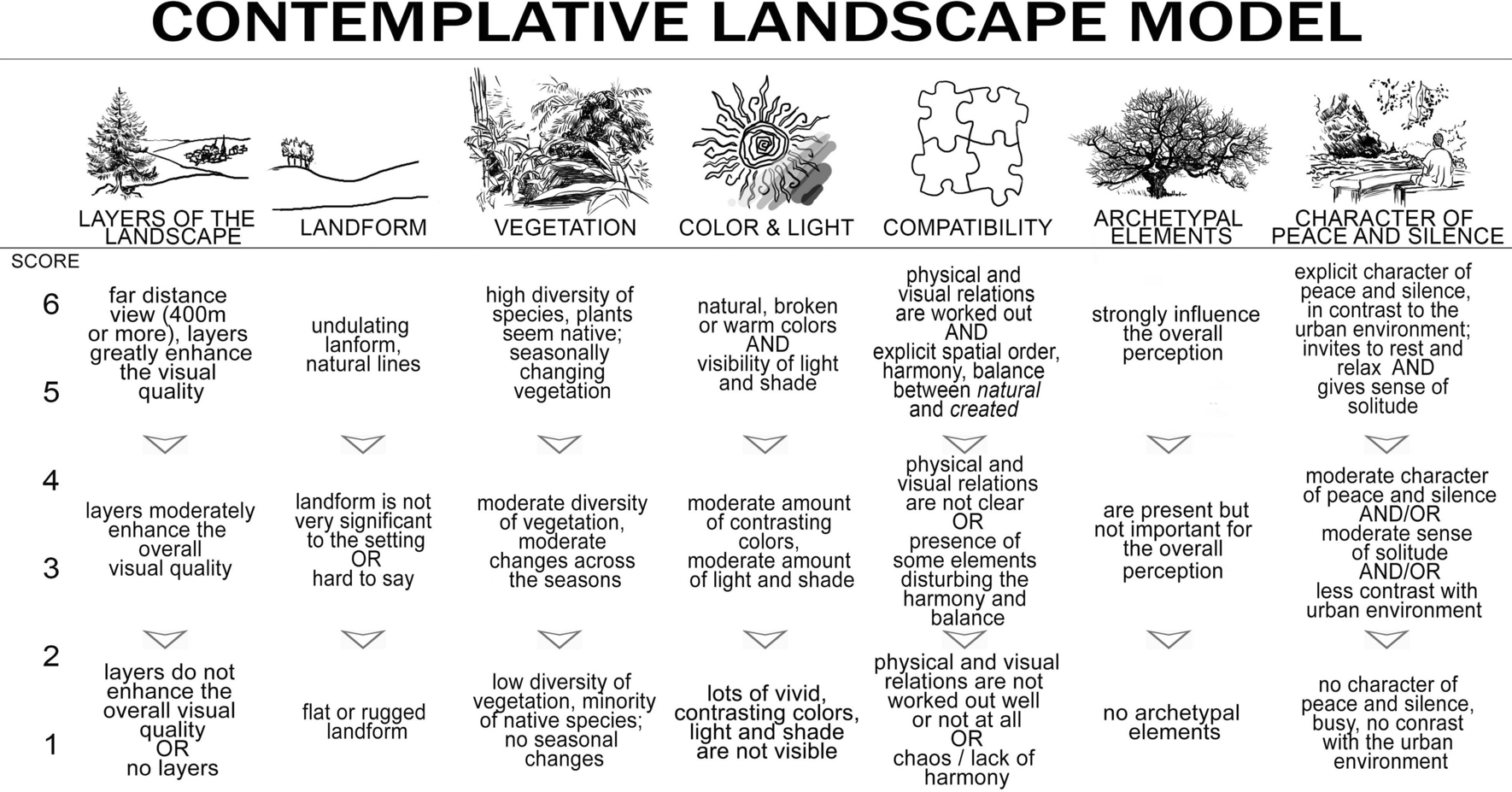This image depicts a detailed table labeled "CONTEMPLATIVE LANDSCAPE MODEL" at the top in large black text. Below, the table is organized into seven columns, each with a header, icon, and descriptive labels: "Layers of the Landscape" featuring a pine tree, "Landform" with tiny trees, "Vegetation" illustrated with plants, "Color and Light" accompanied by a sun drawing, "Compatibility" symbolized by puzzle pieces, "Architectural Elements" represented by a tree, and "Character of Peace and Silence" showing a meditative figure by water. Each column contains a flow chart, which describes the layers and their influence on visual quality. The rows are scored from 6 (highest) to 1 (lowest). The "Layers of the Landscape" column categorizes various elements, including flat or rugged landform, and undulating natural lines. Under "Vegetation," it mentions low to high diversity levels and the presence of native species. The chart explains how increasing layers, particularly in landform, vegetation, and compatibility, enhance the overall visual quality, with detailed levels describing minimal to moderate enhancement across the rows.